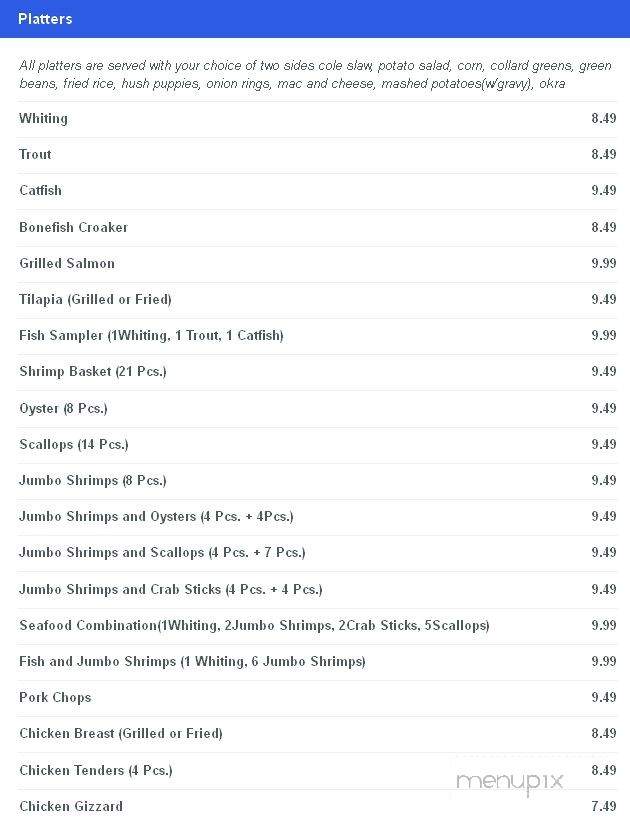"Introducing our platter selection, where every meal is paired with your choice of delectable sides, including potato sides, coleslaw, corn, collard greens, green beans, fried rice, hushpuppies, onion rings, mac and cheese, mashed potatoes, and grated okra. 

1. **Fish Platters**:
   - Whiting ($8.49)
   - Trout ($8.49)
   - Catfish ($8.49)
   - Bonefish ($8.49)
   - Koker ($8.49)
   - Salmon ($9.99)
   - Tilapia ($9.49)

2. **Seafood Baskets**:
   - Shrimp Basket (20 pieces) - $9.49
   - Oyster Basket (8 pieces) - $9.49
   - Scallop Basket (14 pieces)
   - Jumbo Shrimp Basket (8 pieces) - $9.49
   - Jumbo Shrimp Basket (4 pieces)

3. **Mixed Seafood Platters**:
   - Jumbo Shrimp and Scallops (4 pieces shrimp & 7 pieces scallops)
   - Jumbo Shrimp and Crabs (6 jumbo shrimp and 4 crabs)
   - Seafood Combination: 1 Whiting, 2 Jumbo Shrimp, 2 Crabs & 5 Scallops
   - Fish and Jumbo Shrimp: 1 Whiting, 6 Jumbo Shrimp

4. **Chicken Options**:
   - Chicken Breast
   - Cod Fry (2 containers)
   - Chicken Gizzard ($7.49)

Each platter guarantees an array of flavors and textures designed to satisfy your seafood cravings. Enjoy a hearty, well-rounded meal with our extensive selection of sides and main courses."